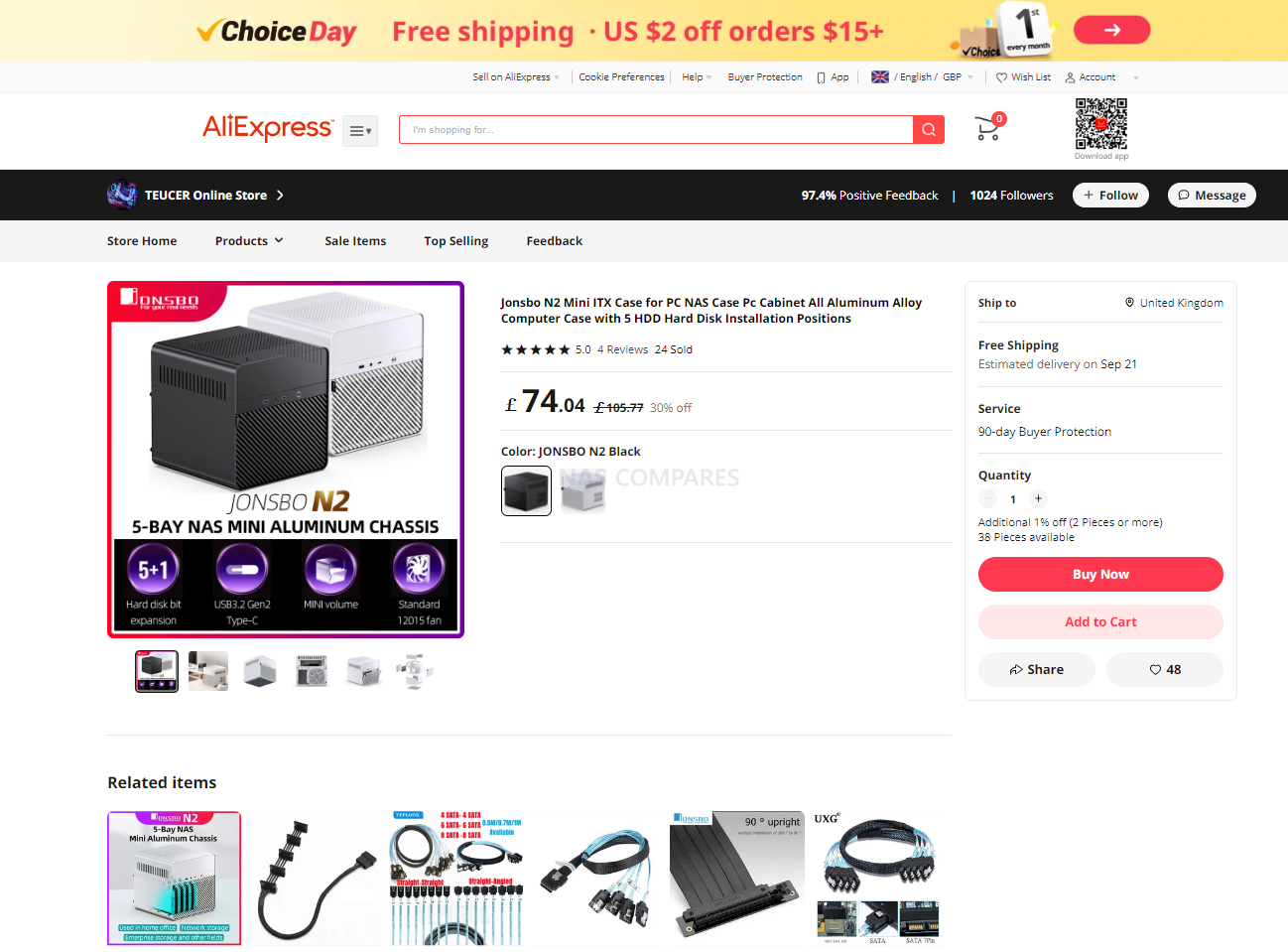**Detailed Caption for AliExpress Website Screenshot**

The screenshot captures the AliExpress website, with a prominent yellow banner at the top announcing "Choice Day" promotions, including free shipping and a discount of $2 off orders over $15. Just below the banner, a navigation bar offers links to "Sell on AliExpress," "Cookie Preferences," "Help," "Buyer Protection," "App," "English," "GBP," "Wish List," and "Account."

Centered on the page is the AliExpress logo accompanied by a search bar labeled "I am shopping for..." with a red search icon on its right. A shopping cart icon shows a count of zero items, and there is also a QR code available for app downloads.

A black border section introduces the "Tucer Online Store," marked with a positive feedback score of 97.4% and 1,024 followers. Follow and message buttons are prominently displayed. The store’s navigation menu lists "Store Home," "Products," "Sale Items," "Top Selling," and "Feedback."

In the main content area, there is an image featuring two versions of a case - one black and one white. The listing title reads "Jonesbow N2 Mini ITX Case for PC NAS Case, PC Cabinet, All Aluminum Alloy Computer Case with 5 HDD Hard Disk Installation Positions." The price is listed as £74, with the black version selected by default. Information about free shipping and an estimated delivery date of September 21st is provided, alongside reassurance of buyer protection. Options to adjust the quantity, and buttons labeled "Buy Now," "Add to Cart," and "Share" are available. A heart icon, indicating the number of people who have liked this item, shows the number 48. Below the main product, there are images of related items.